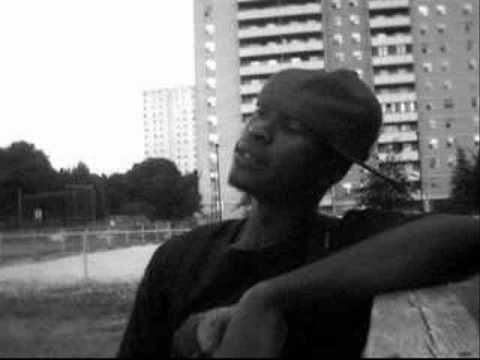In this detailed black and white photograph, we see an African-American man standing at the center of the frame, gazing intently into the distance towards the left side of the image. He is clad in a dark-colored t-shirt and wearing a backwards baseball cap. His posture is composed, with his left arm resting on a wooden platform, identifiable by a prominent crack running through it. The man, who appears to be in his 20s to 40s, has his chin slightly raised, lips parted to show a glimpse of his teeth, and eyes half-closed, giving him a serene, reflective expression.

In the background, a large building towers immediately behind him, with another structure further off to the left, suggesting a cityscape dotted with apartment complexes or skyscrapers featuring numerous windows and balconies. Adding to the scenic backdrop are several trees and a metal fence, possibly bordering a field of dirt or grass, contributing to the urban yet somewhat pastoral ambiance.